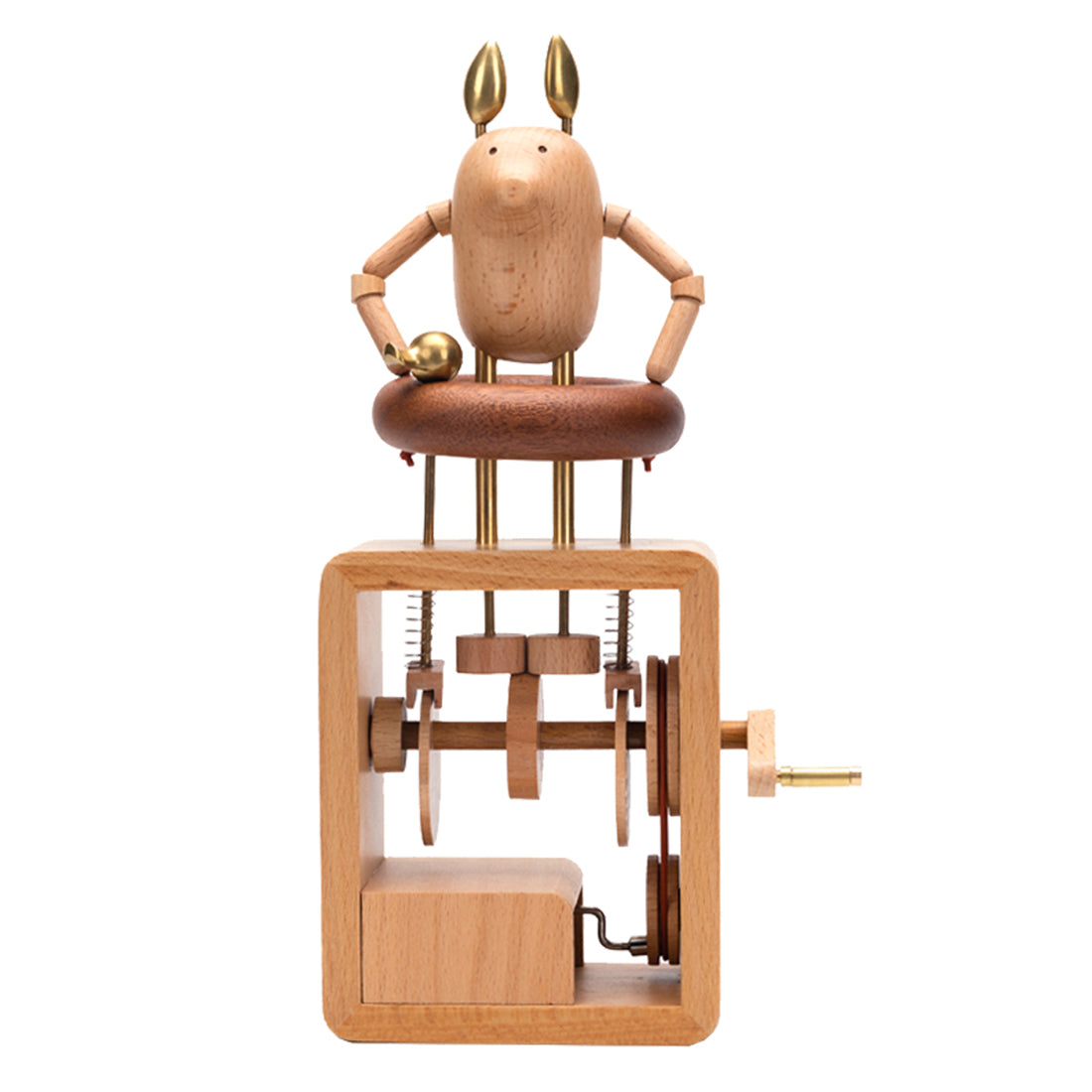This intricate wooden contraption resembles a whimsical, handcrafted toy, taking the form of a pig with beady black eyes and golden ears. The pig stands atop the device, holding a golden bell in its left hand. The body of the contraption, crafted from light brown carved wood, contains wooden gears, shafts, and circles intricately connected by strings and pulleys. The pig's legs are slender golden pins extending downward into the middle of the box. There is a crank on the right-hand side; when turned, it likely activates the inner workings, lifting the bell in the pig's hand and prompting it to ring. This pig figure, seemingly made from various carved wooden pieces, is an endearing centerpiece, adding charm to the mechanism which combines the nostalgic feel of a music box with the playful surprise element reminiscent of a jack-in-the-box.